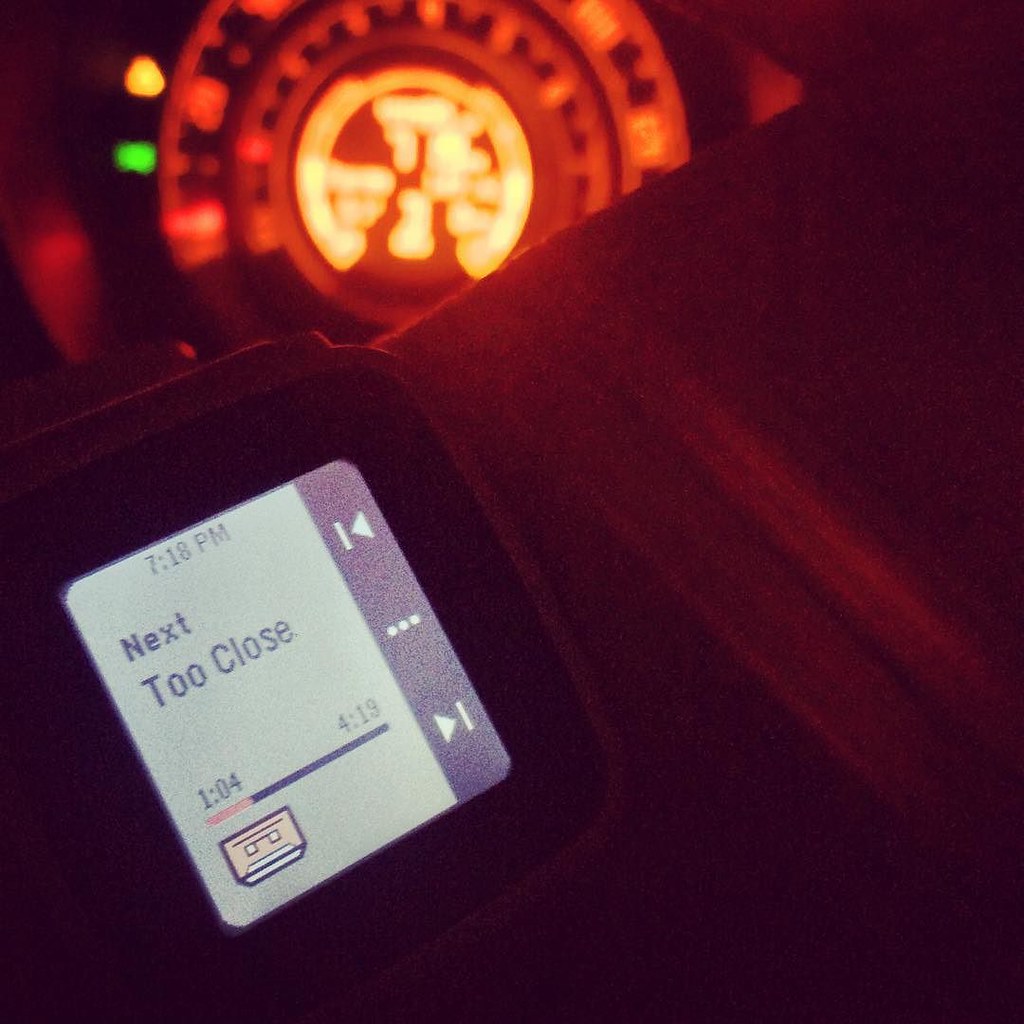The image is a large, square composition where most of the background is heavily blurred, creating a mysterious, diffuse ambiance. Dominating the upper portion is a circular dial that is brightly illuminated with a combination of yellow and orange lights, casting a warm, glowy aura around its edges. The intricate designs within the dial are bathed in a yellowish-orange light that draws the eye, but details remain indistinct due to the blurriness. Below this, a shadowy brown surface extends downward, though its features are not clearly discernible.

In the lower left corner of the image, prominently displayed, is a digital screen that closely resembles an Apple smartwatch, with its signature rounded rectangular shape. The screen gleams in white and gray hues, displaying the time as 7:18 PM at the top. On the left side of the screen, it reads "next" and "too close," while a segmented bar at the bottom reveals the numbers "1.04" on the left and "4,19" on the right, likely indicating a progress tracker. Along the right edge of the screen are iconographic fast forward and reverse symbols, reinforcing the idea that this is a music player interface. All these elements together create a vivid yet enigmatic scene, dominated by glowing light and digital intricacies.